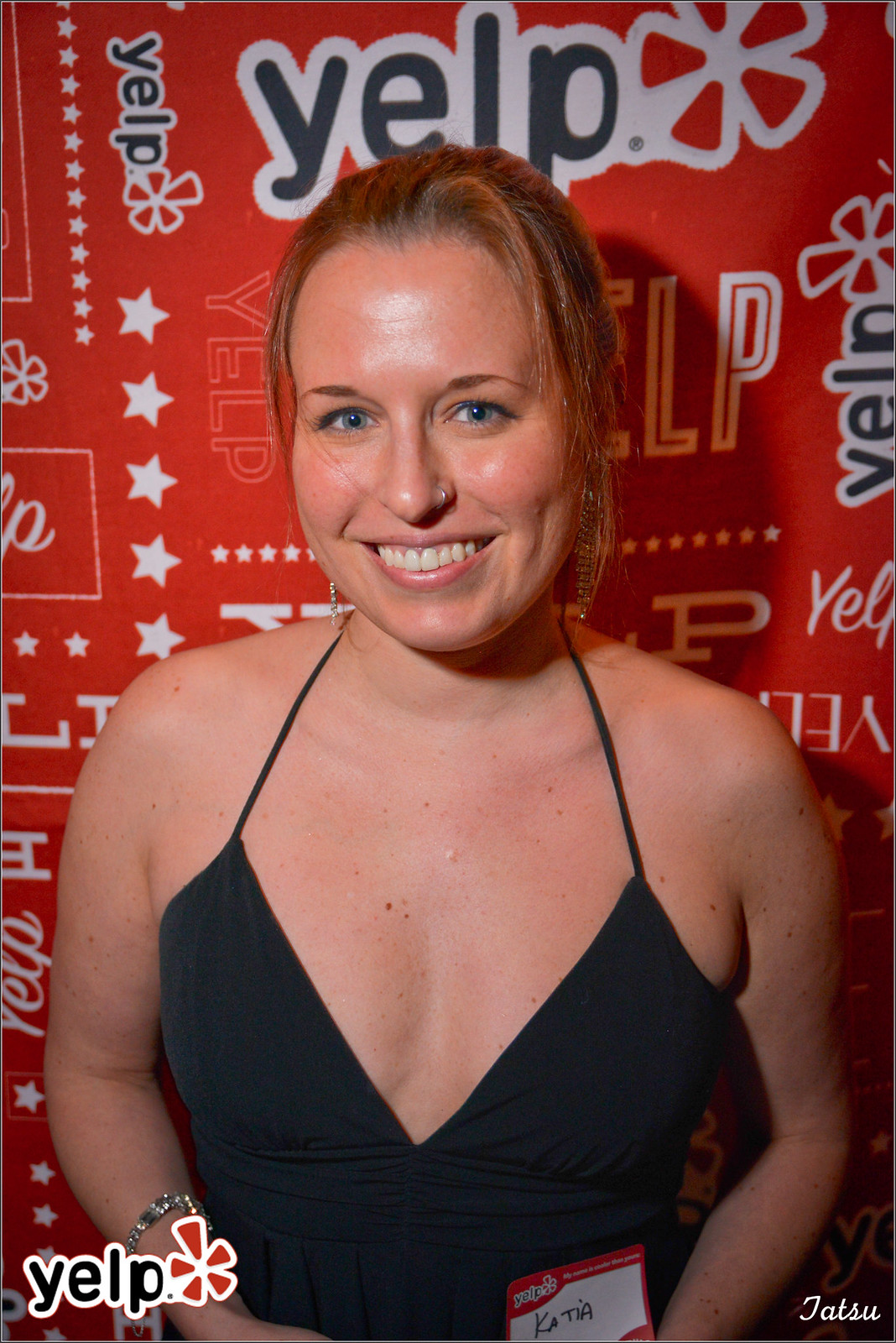The photograph captures a woman named Katia, as indicated by the white name tag with a red border affixed to her black dress with thin straps. She has chin or shoulder-length blonde hair, blue eyes, a nose piercing on her left nostril, and appears to be smiling at the camera. She sports a sparkly bracelet on her right wrist and shiny dangly earrings. The backdrop is a red board with various renditions of the Yelp logo—both text and abstract flower-shaped symbols—suggesting she’s at a Yelp event. In the bottom left corner, there is another Yelp logo, while the bottom right corner includes the text "Tatsu."